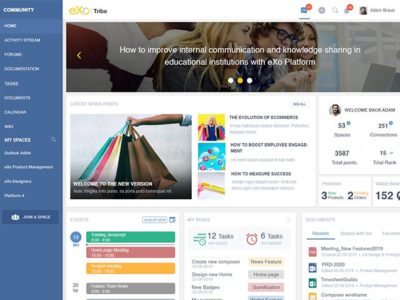The image depicts a website identified as EXO Tribe, tailored specifically for educational institutions such as schools, universities, and other teaching platforms. At the top of the website, there's a prominent header advertisement stating, "How to improve internal communication and knowledge sharing in educational institutions with EXO platform," indicating the platform's emphasis on enhancing communication and collaboration within these settings. Though the snapshot is somewhat blurry, making fine details difficult to discern, several functionalities of the site are visible.

On the main interface, you'll find an option for viewing tasks, coupled with a calendar layout for scheduling and organizational purposes. An image of a person holding multiple bags is shown with a caption below stating, "Welcome to the new version," suggesting that the website has recently undergone an update. The left-hand side menu provides various navigation options, starting with 'Community' at the top, followed by 'Home' and several other links for different pages within the site.

In the top right-hand corner, there's an image icon and an individual’s name, likely serving as a shortcut to the user’s profile settings and personal information. Despite the blurriness, the layout and features point towards a user-friendly, updated platform aimed at fostering better internal communication and knowledge sharing in educational environments.